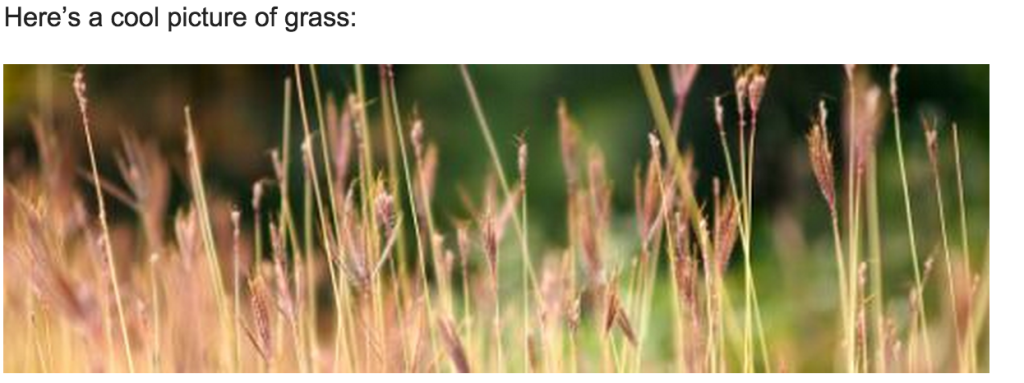This detailed, close-up photograph features an elongated rectangle of grass blades, presented beneath a black Arial font caption reading "Here's a cool picture of grass" on a white background. The picture reveals numerous thin and delicate strands of grass stretching across the entire horizontal frame, with a concentration of blades more densely packed on the left side. The left and central sections predominantly display dry, brown, and occasionally purplish-hued grass, with some tips exhibiting a faint pink blend. This contrasts with the right section, where the grass appears slightly taller and greener, suggesting different stages of growth or health. The tops of many brown blades are fuzzy, branching into fine, needle-like endings. The blurred, wooded background, blending greens and browns, enhances the focus on the intricate details and varied colors of the grass, evoking a late spring to fall atmosphere.